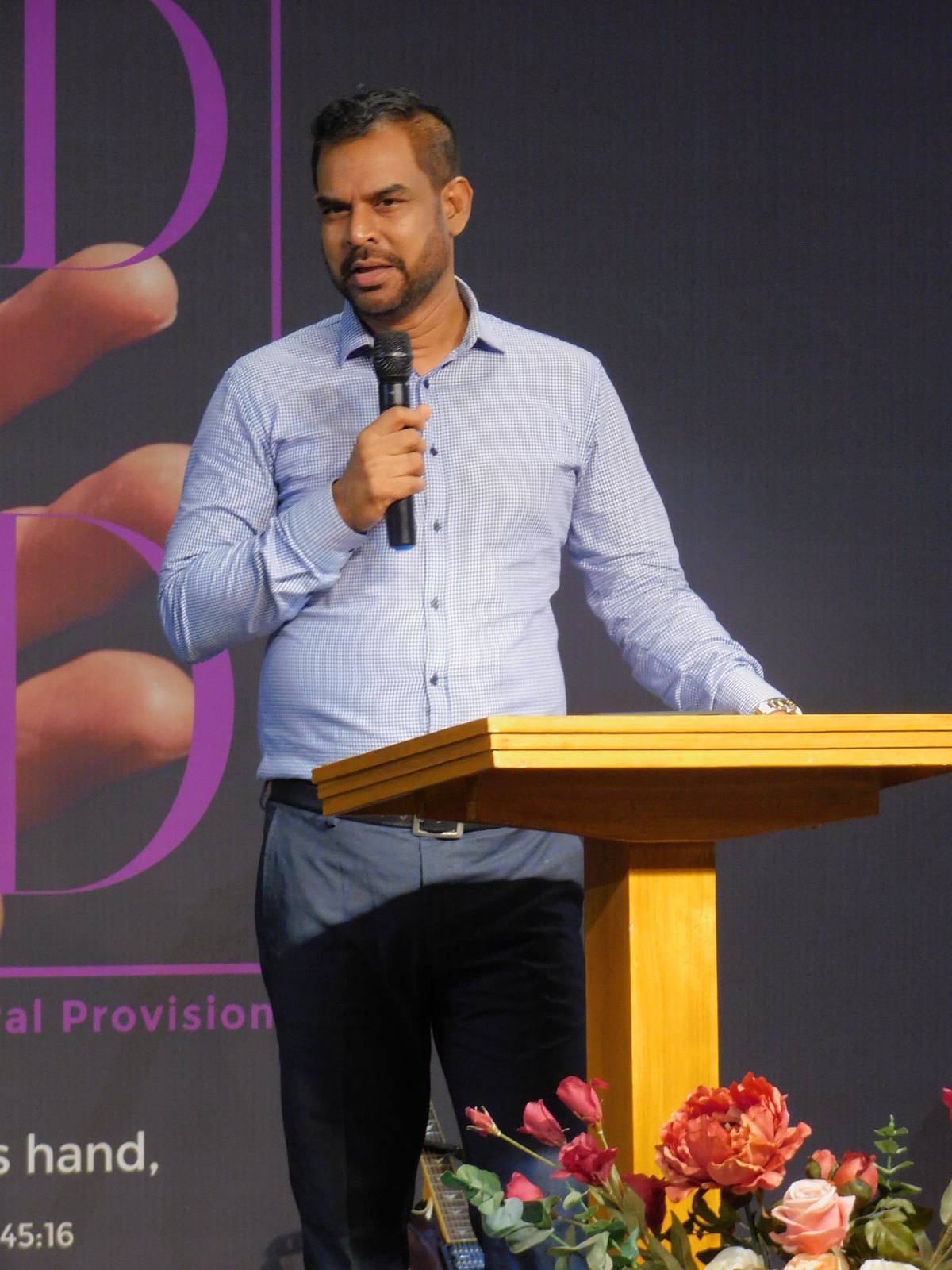The image shows a rectangular photograph of a well-dressed man addressing a crowd from a stage. He stands behind a light brown wooden podium with distinctive wood grains, one hand resting on it, adorned with a silver wristwatch. In his other hand, he holds a black microphone. The man is light-skinned, with short dark hair shaved on the sides, and a neat beard and mustache. He wears a blue and white checkered button-up shirt with black buttons and a collar, paired with gray dress pants, a black belt, and a silver buckle. In front of the podium is a bouquet of mixed flowers featuring red and pink roses, peonies, and other assorted blooms with some greenery, suggesting an artificial arrangement. The backdrop is a solid black with a superimposed image of a hand and the partially visible letters "D" in purple, the word "provision," and other obscured text including "hand" in white and "45, 16." The setting appears to be indoors, perhaps during a presentation or lecture, with the man centered in the image and the flowers positioned in the bottom right corner.